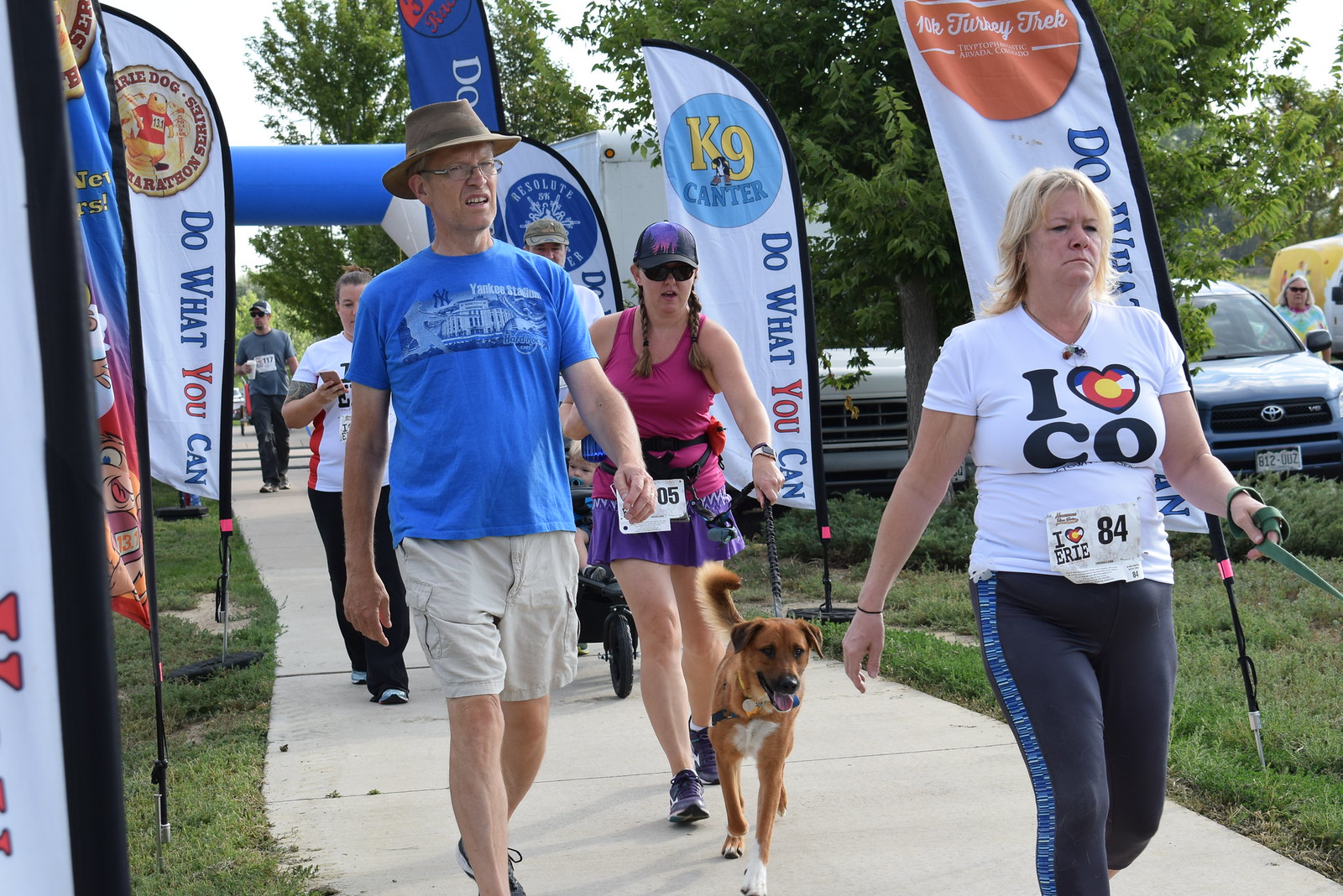The photograph captures a lively scene from a marathon or walk-a-thon with participants moving along a large, white concrete sidewalk segmented into small sections. On either side of the path, vibrant green grass frames the walkway, adorned with uniform white flag banners mounted on black poles, each proudly displaying different logos alongside the encouraging mantra, "Do What You Can." 

In the foreground, a woman stands out, sporting blonde hair and wearing black pants with a blue stripe and a white V-neck shirt branded with "I ❤️ CO," where the heart features a red "C." She is holding a leash, guiding her through the event. Affixed to her front is a number tag that reads "I ❤️ Erie 84."

Following closely behind her, a man is dressed in a blue shirt, brown brimmed hat, cargo shorts, and glasses. Further back, there's a woman decked out in a pink tank top with a purple skirt, holding a brown dog walking in front of her. She completes her outfit with a black hat. Additional participants can be seen trailing behind these front runners, filling the scene with a sense of community and shared motivation. To the far right of the image, a parking lot with numerous parked cars is visible, indicating the event’s significant turnout.